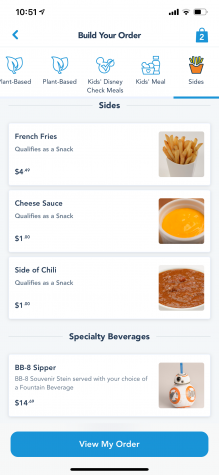This image is a screenshot from a mobile food-ordering app, likely used at Disneyland. The screenshot captures the "Build Your Order" section, showcasing the "Sides" category along with a specialty beverage. The available sides include:

1. **French Fries** - Priced at $4.99 and categorized as a snack, depicted as a small container of crispy fries.
2. **Cheese Sauce** - Priced at $1.00, also a snack, represented by a small bowl of yellow cheese sauce.
3. **Side of Chili** - Priced at $1.00 and categorized as a snack.

In addition to these sides, the app features a specialty beverage:

- **BB-8 Sipper** - A souvenir sipper priced at $14.99, which includes your choice of fountain beverage. It is designed to resemble the BB-8 droid from the Star Wars franchise, functioning as a unique drinking container.

The screenshot appears to highlight the stark contrast in pricing between a modest dollar-side of cheese and the considerably more expensive BB-8 sipper, emphasizing a sense of amusement or frustration at the perceived price inflation typical in theme parks like Disneyland. The app also suggests it is at Disney by noting the plant-based options and Kids Disney Check Meals in the menu.